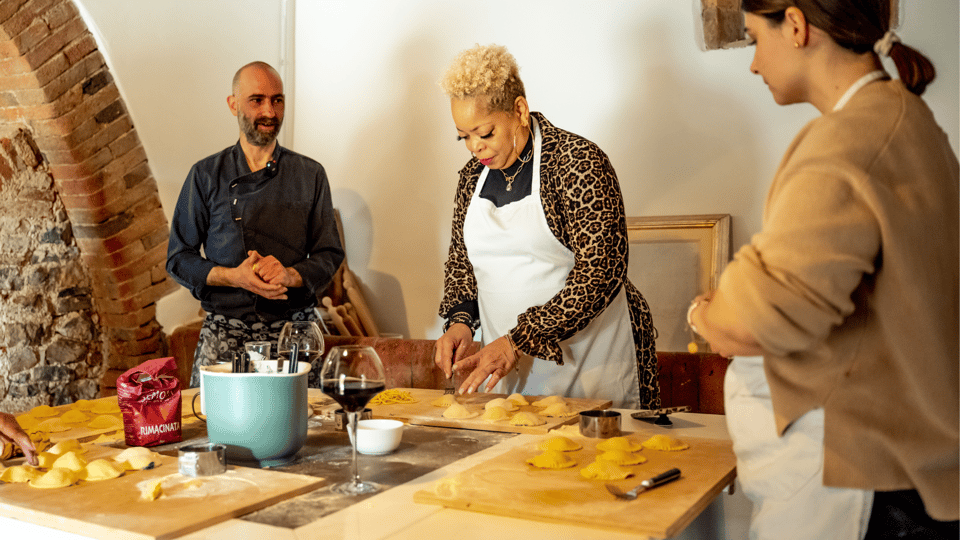In this detailed photograph set in a kitchen with white walls and an arch made of red bricks on the left, three individuals are engaged in a culinary activity, likely a cooking class. On the right, a woman with black hair pulled back into a ponytail wears a brown jacket under her white apron and appears to be pregnant. In the center, an older woman with dark skin and blonde hair dons a leopard print, long-sleeved shirt and a white apron. Both women focus on their cutting boards, which are topped with yellow dumplings that resemble ravioli. In front of them is a blue bowl and wine glasses filled with red wine. A bald man with a beard and a black button-up shirt stands in the background to the left, possibly the instructor given his observational stance. The room also contains various cooking utensils, a big seafoam green pot, and a red bag. A picture frame with a silver border leans against the wall, hinting at the cozy, homely environment.